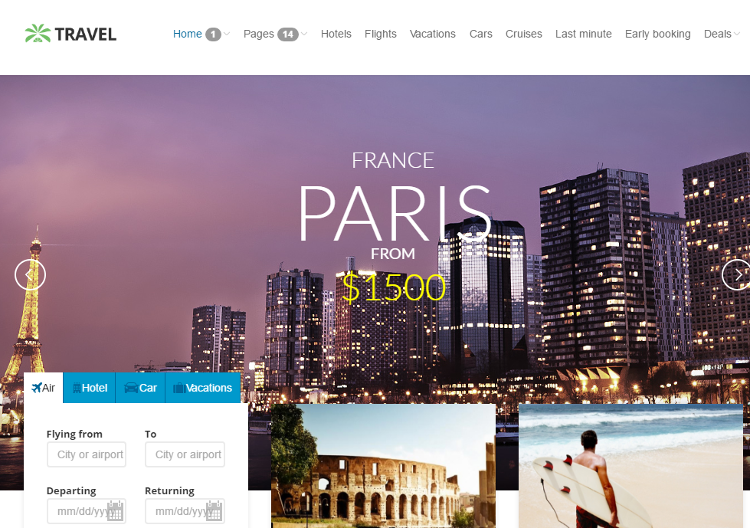This image is a detailed screenshot from a travel website. In the upper left-hand corner, the site’s logo, featuring a stylized palm tree, is positioned next to the word "Travel." The navigation bar at the top includes various menu options: Home, Pages, Hotels, Flights, Vacations, Cars, Cruises, Last Minute, Early Booking, and Deals. 

Occupying the main section is a prominent photograph displaying the iconic Eiffel Tower on the left and a cluster of Parisian buildings on the right, accompanied by the text "France Paris from $1,500." 

In the bottom left corner, a section offers options for Air, Hotel, Car, and Vacations, currently displayed on the Air tab. Here, users are prompted to enter details for flying from and to, with fields for departing and returning dates. 

To the right of this section, there are two additional photographs. The central photo captures the exterior of a famous architectural landmark, while the far-right image depicts a serene beach scene, featuring an individual walking with a surfboard in hand.